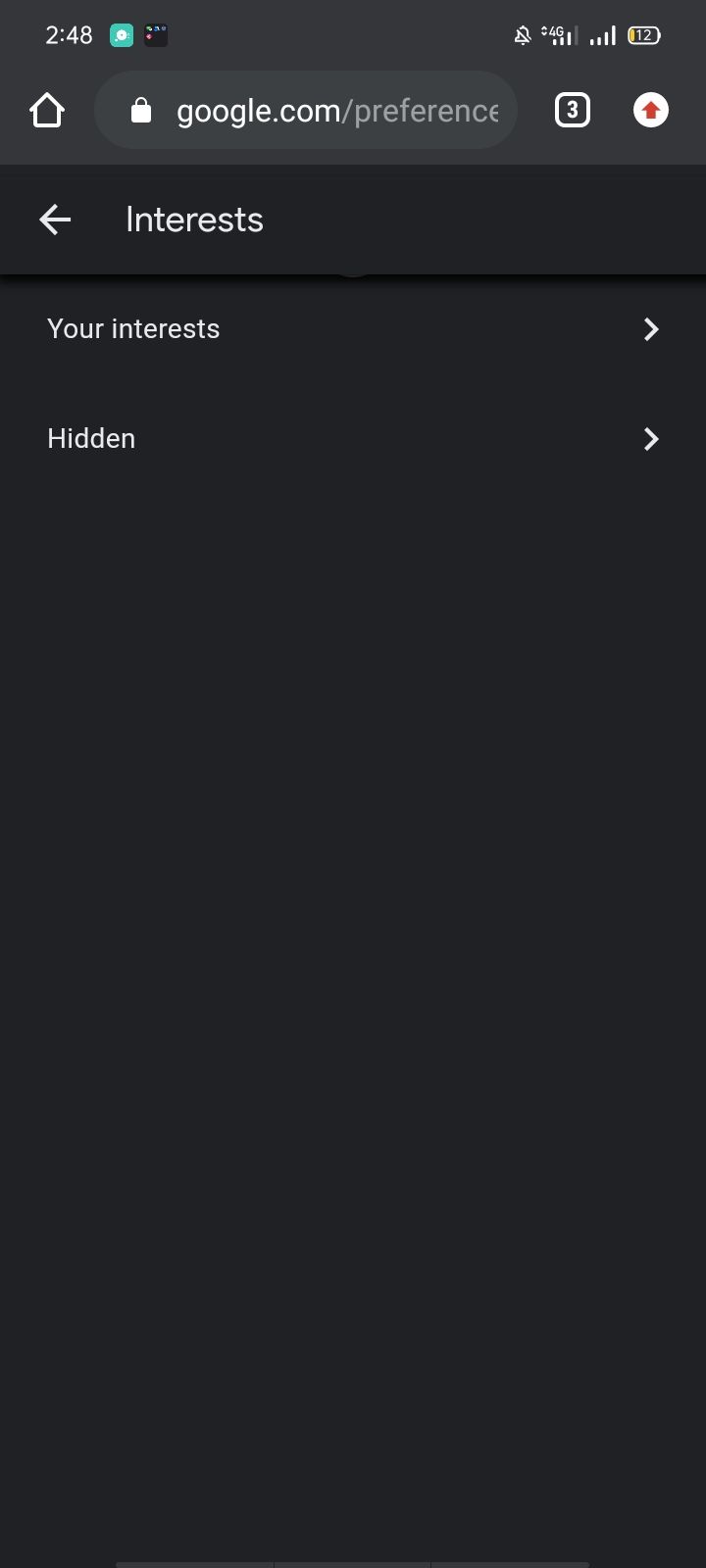Screenshot depicting a dark-themed user interface, showing the battery level at 12% with 248 notifications. The screen displays the URL "google.com/preferences" with a home icon beside it. In the center, a square labeled with the number "3" is prominently featured. A white circle contains a red upward-pointing arrow, indicating an increase or ascent. The section labeled "Your Interests" features an arrow pointing left towards "Interests," and to the right of "Hidden," there is another arrow pointing right.